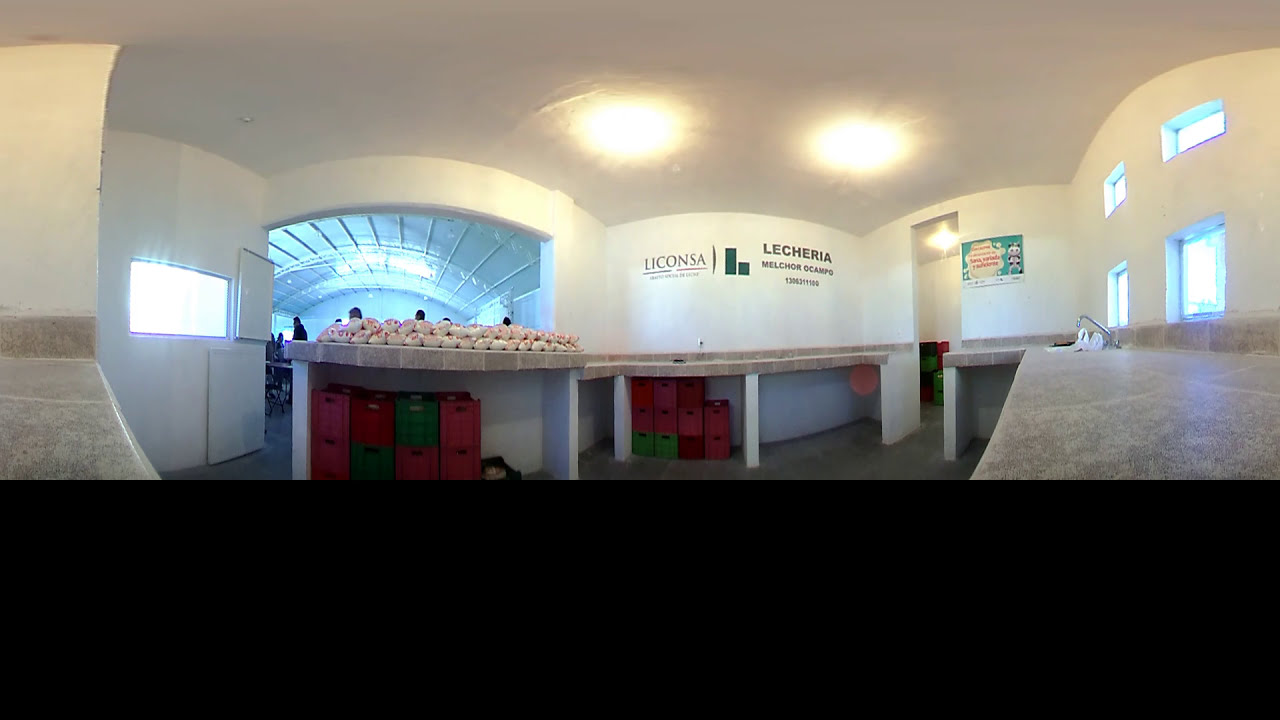The digital photograph depicts the interior of an industrial-style kitchen or market, set indoors during the day. The image is filled with vibrant colors, including white, yellow, light blue, red, green, tan, and black. The layout is spacious but lacks a central focus, with various elements scattered across the frame.
At the bottom of the image, a black banner or border runs across the screen. To the right, a sink is visible alongside a countertop cluttered with dozens of small plastic bags. Windows and doorways are present, revealing multiple sections of the building, some topped with a curved, dome-like roof.

Behind the counter, there are crates of different colors stored, hinting at an organized storage area. Above, lights hang from the ceiling, illuminating the setting. In front of the frame, a little stand displays white objects, possibly merchandise for sale, with additional plastic containers underneath. The exact nature of some items remains unclear due to the text being illegible, possibly because it is in a different language or too small to read. The overall ambiance suggests a busy, functional space, potentially a market or food preparation area, filled with practical storage solutions and vibrant activity.